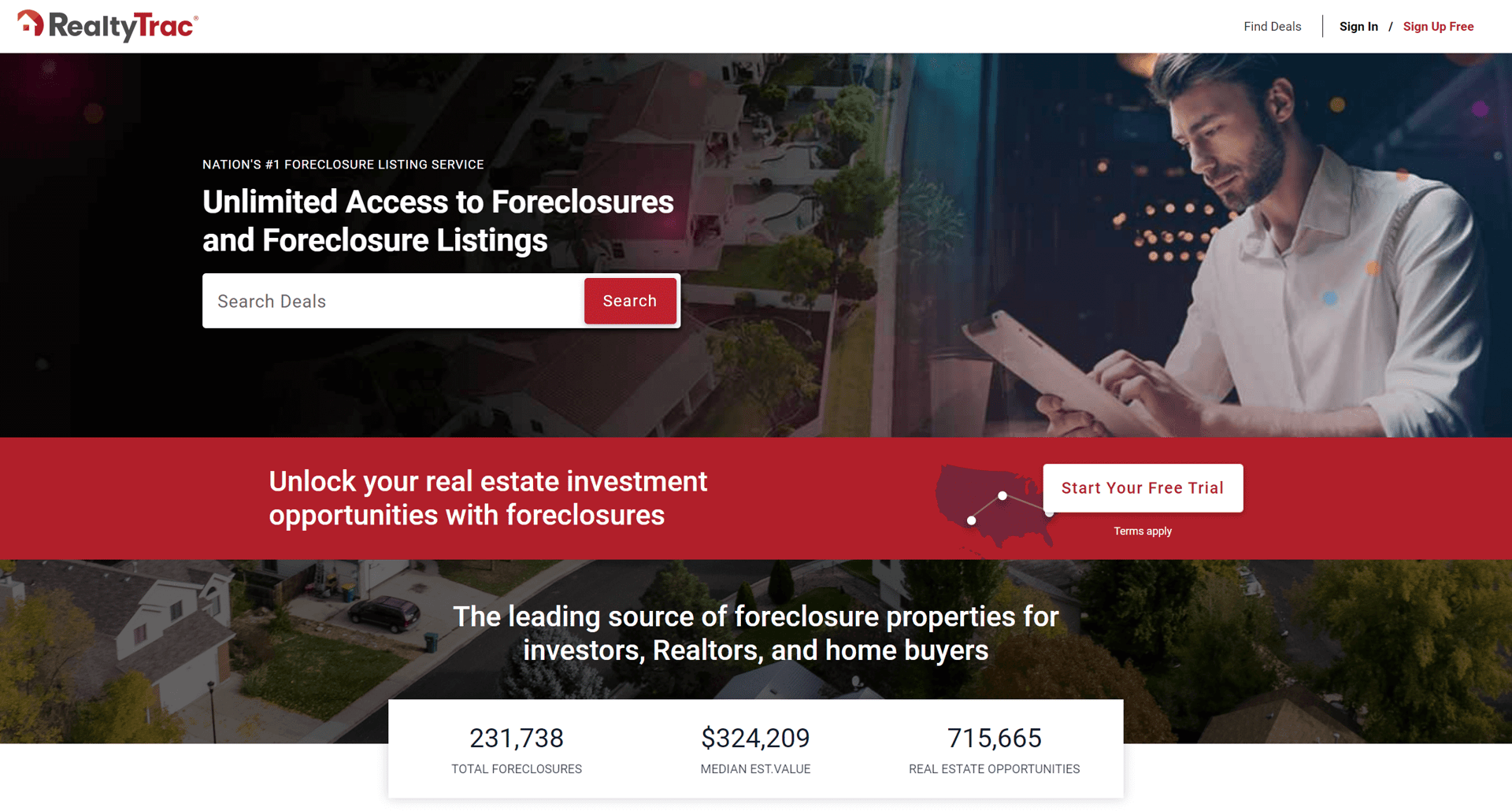The screenshot depicts the first half of a real estate investment landing page. The background features a silhouette of a neighborhood that transitions into an image of a man using an iPad set against an urban landscape. In bold, white text, the landing page advertises "Unlimited access to foreclosures and foreclosure listings," emphasizing the opportunity for users to search for deals. A prominent red banner spans the width of the page, stating, "Unlock your real estate investment opportunities with foreclosures." Below this is an illustration of the United States alongside a white button inviting visitors to "Start Your Free Trial." Further down, the page asserts its status as the "leading source of foreclosures," providing specific data such as the number of foreclosures, the median property value, and various real estate investment opportunities. This landing page is clearly designed to attract investors seeking information and access to foreclosure properties.